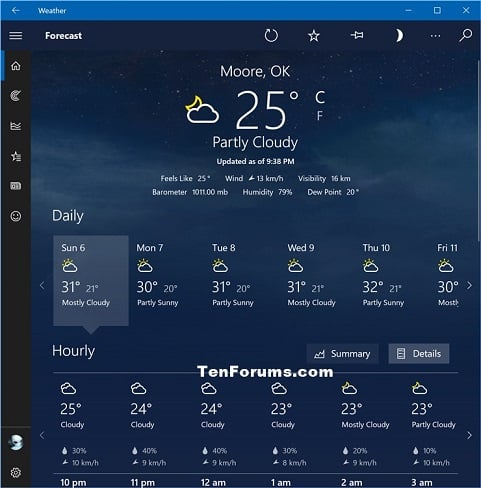**Detailed Weather App Screenshot Description:**

At the top left corner of the main page, a header in blue background with white text prominently displays the word "Weather." Below this, a secondary header in purple background carries the title "Forecast" on the top right.

A sidebar menu on the left features a black background with highlighted icons poised for selection. On the top right of the screen, several white tabs labeled "Refresh," "Favorite," "Pin," "Night Mode," "Options," and a search icon are visibly positioned.

In the center of the display, comprehensive weather details for a specific city are presented. It reads, "25°C, Partly Cloudy, updated at 9:08 PM." Additional weather metrics include "Feels like 25°C," wind speed of "10 km/h," visibility of "16 km," barometric pressure of "1010.0 mb," humidity at "79%," and a dew point of "20%."

A daily weather forecast follows:
- **Sunday:** High of 31°C, Low of 21°C, mostly cloudy.
- **Monday:** High of 30°C, Low of 20°C, partly sunny.
- **Tuesday:** High of 31°C, Low of 20°C, partly sunny.
- **Wednesday:** High of 31°C, Low of 21°C, mostly cloudy.
- **Thursday:** High of 32°C, Low of 21°C, partly sunny.
- **Friday:** High of 32°C, Low of 21°C, partly sunny.

An hourly weather forecast for the night:
- **10 PM:** 25°C, cloudy.
- **11 PM:** 24°C, cloudy.
- **12 AM:** 24°C, cloudy.
- **1 AM:** 20°C, cloudy.
- **2 AM:** 20°C, mostly cloudy.
- **3 AM:** 20°C, partly cloudy.

The background of the app depicts a night sky scene, characterized by a dark blue gradient with dark grey clouds and subtle star elements.